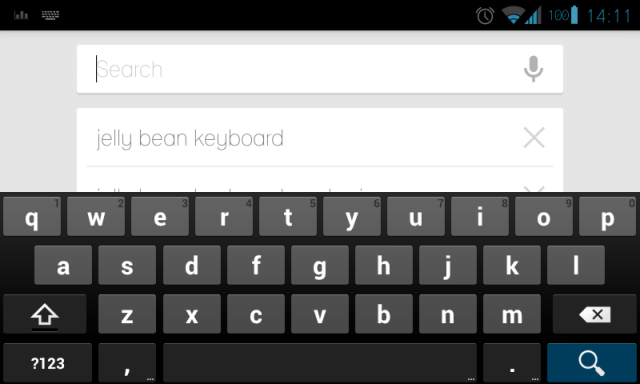The screenshot captures a horizontally oriented Android phone screen. In the top left corner of the status bar, there are two icons: a small menu icon comprised of three horizontal lines and a keyboard icon. On the right side of the status bar, there's an alarm clock icon indicating an active alarm, followed by a Wi-Fi icon with two blue lines of coverage and a mobile data icon showing three blue bars of signal strength. The battery icon displays a full charge at 100%, and the current time is 2:11 PM.

Below the status bar, a search bar is prominently displayed with faint, placeholder text reading "search.” On the right side of the search bar, there is a microphone icon for voice search functionality. Beneath the search bar, a suggested search option for "Jelly Bean Keyboard" is visible, along with an active keyboard interface, implying that the user may be exploring alternative keyboards or keyboard customization options for their Android device.